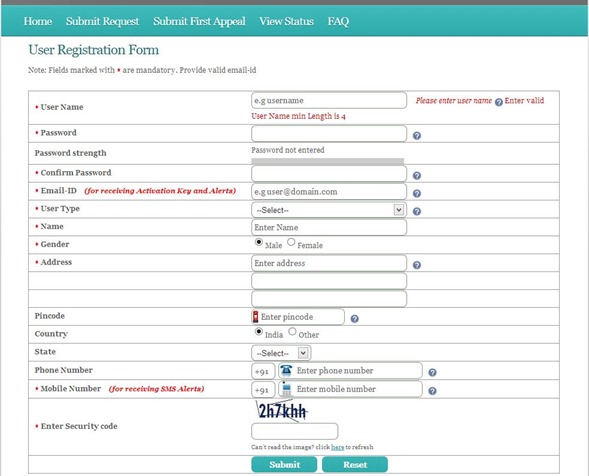A detailed screenshot of a user registration form displayed on a digital device such as a PC, laptop, or tablet. The top of the image features a turquoise blue navigation bar with white text listing options: "Home," "Submit Request," "Submit First Appeal," "View Status," and "FAQ." Below this bar, on a white background, the title "User Registration Form" is prominently displayed. The form contains numerous labeled fields with corresponding text boxes for user input.

Fields marked with a red asterisk are mandatory, with a note highlighting the necessity of providing a valid email ID. From top to bottom on the left side of the form, the labels are as follows: Username, Password, Password Strength, Confirm Password, Email ID, User Type, Name, Gender, Address, PIN Code, Country, State, Phone Number, Mobile Number, and Enter Security Code. Positioned to the right of the "Enter Security Code" label is a typical CAPTCHA featuring both alphanumeric characters, accompanied by an empty text box underneath for user entry. 

At the bottom of the form, beneath the CAPTCHA box, there are blue buttons with white lettering for "Submit" and "Reset" actions. The right-hand side of the form shows each label with its corresponding empty text box, awaiting user input as the form is to be filled out.